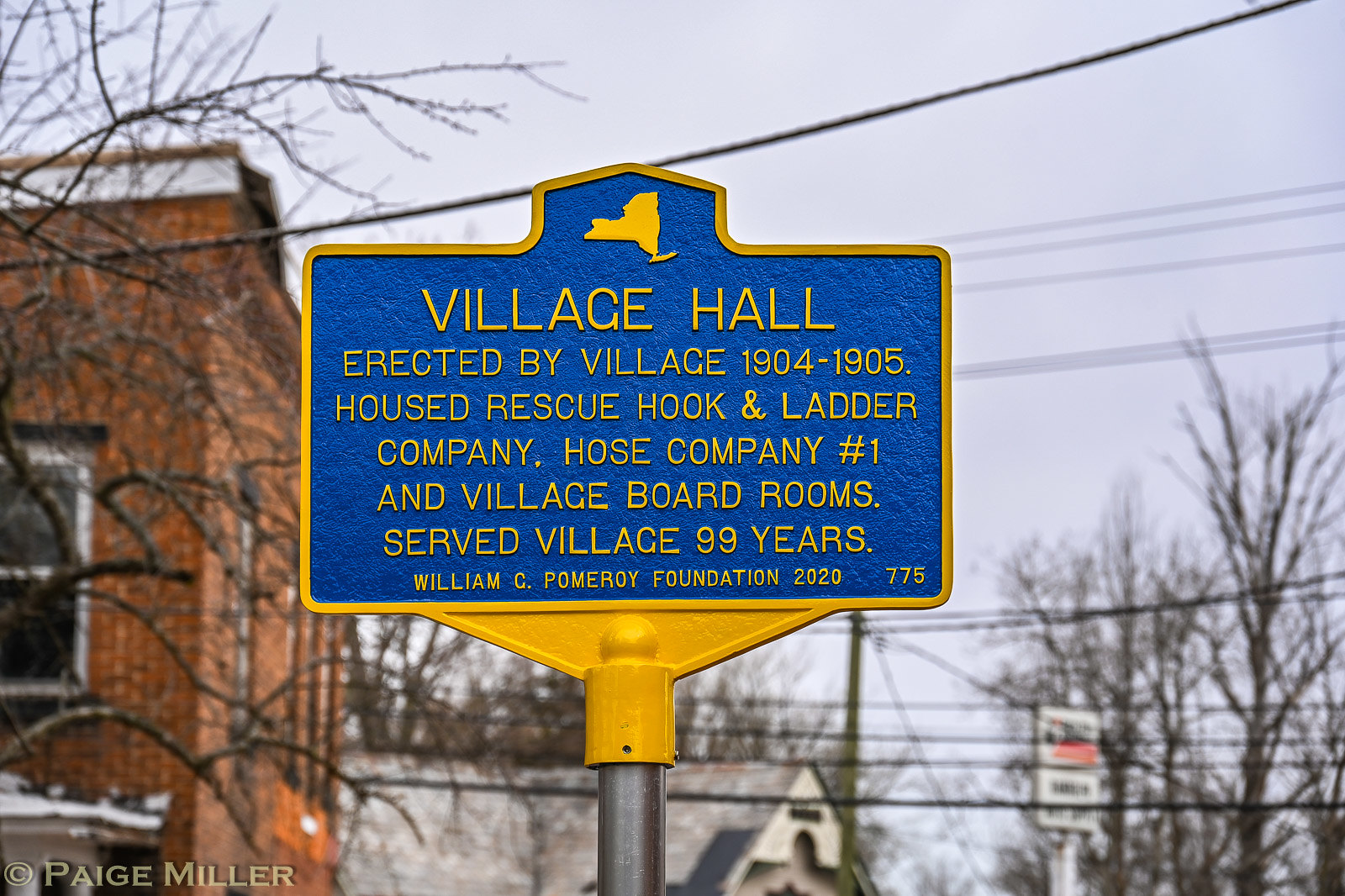This image captures an outdoor setting during daytime, featuring a detailed historical sign prominently displayed in the center. The sign is crafted from metal and painted royal blue, with a creatively designed orange border. At the top center of the sign is a small emblem resembling the state of New York in yellow. The text on the sign reads: "Village Hall, erected by Village 1904-1905. Housed Rescue Hook and Ladder Company, Host Company No. 1, and Village Board Rooms. Served Village 99 years. William C. Pomeroy Foundation, 2020," with the number 775 in the bottom right corner. In the background, there are various brick buildings, some with large colored walls and glass windows bordered in white, alongside dried trees and sky partially filled with clouds. Electrical wires stretch across the upper part of the image. On the bottom left corner of the sign, the copyright notation "Paige Miller Ward" is visible. The sign stands on a gray pole, contributing to the historical ambiance of the surrounding town street scene.